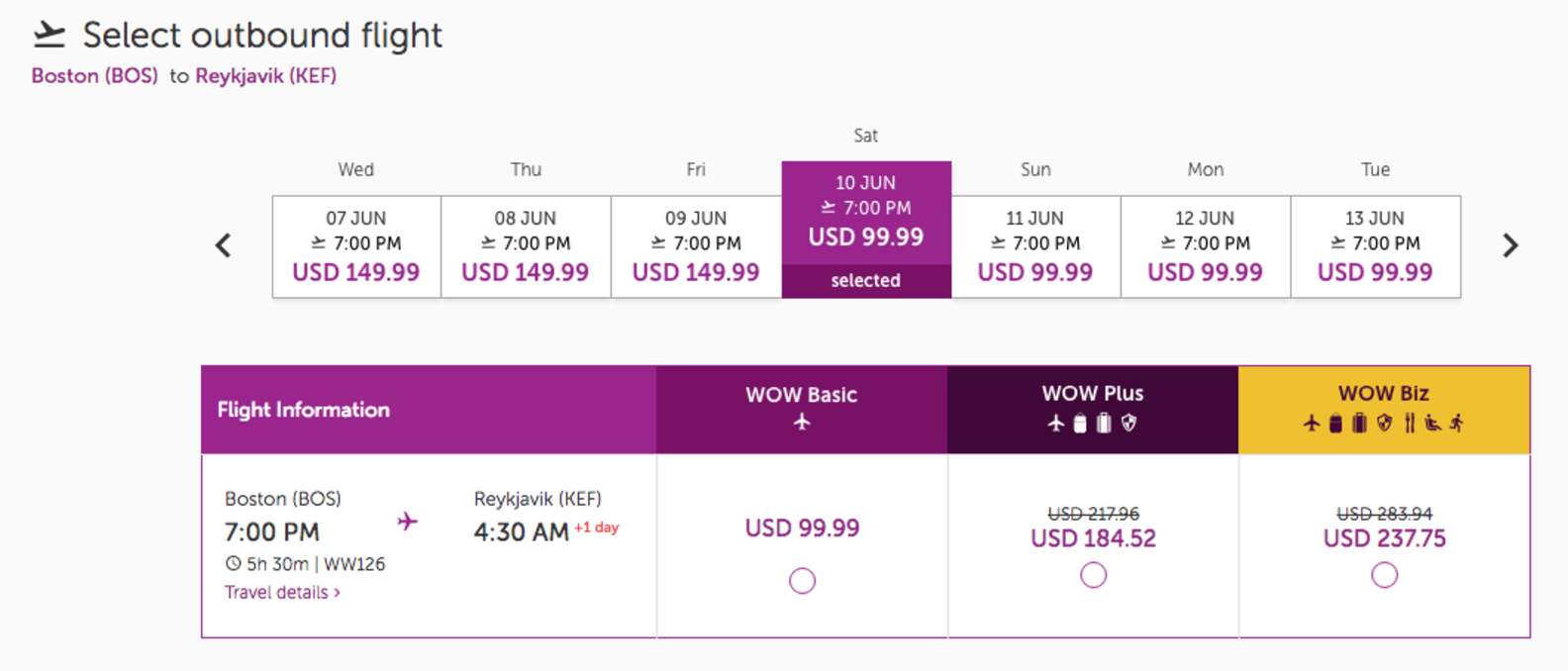This image is a detailed screenshot from an airline booking website. The website appears simplified, without a visible browser bar or identifiable company logo. The top left corner features a minimalistic header: black text reads "Select Outbound Flight," accompanied by a small icon of a plane taking off.

Directly beneath the header, in clickable purple hyperlink text, the departure and destination details are displayed: "Boston BOS to Reykjavik KEF." Below these details, a scrollable calendar spans horizontally from Wednesday to Tuesday, allowing users to navigate through different dates with arrow buttons. The selected date is highlighted in purple: "Saturday, June 10th, 7 p.m. USD 99.99," while other dates remain in a standard white background.

Further down, the site offers three distinct booking options for the selected flight: "WOW Basic" for USD 99.99, "WOW Plus" for USD 184.52, and "WOW Business Class" for USD 237.75, providing additional flexibility and choices for travelers.